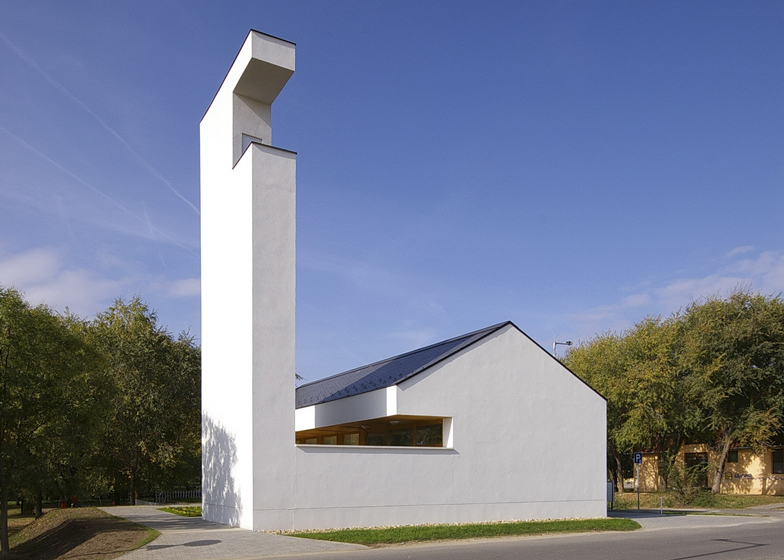The photograph depicts a very peculiar, modern white building under a sunny blue sky with wispy clouds. The structure is situated in a lush, green environment with several trees surrounding it. The building features a typical house shape with a dark-colored, angular, slanted roof but diverges dramatically in design with a large, attached tower that extends twice the height of the building. This tower, protruding from the left side of the house, features a distinctive cut-out "C" shape at the top, reminiscent of a jigsaw piece or an eye. The façade facing the viewer is notably windowless, presenting a stark, blank exterior. A patch of green grass lies in front of the building, complemented by a grey driveway and a street. In the background, a slightly yellow building and a street light can be seen partially obscured by the dense forestry. The environment suggests that the photograph was taken during summer, given the vibrant greenery and the leveling of land presumably done to accommodate the building.